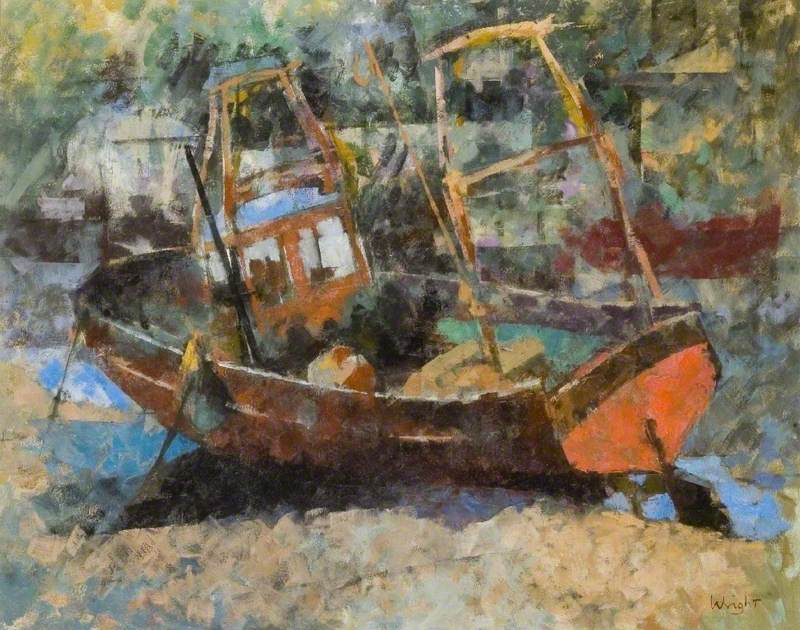This painting depicts a medium-sized, red and brown wooden boat prominently positioned in the center, surrounded by a blue waterway, perhaps a river or lake. The style is impressionistic, characterized by splotches of white and various colors that lend it a blurred yet intentional appearance. The boat has several triangular projections on its sides, with an area that seems to shelter rowers or sailors, potentially used for steering the vessel. The boat's direction and slight lean towards the left are accentuated by the vivid hues and the interplay of light, suggesting a sunny day. The lower portion of the composition features a dirt shore, where the boat's shadow is faintly visible. The background, although faded and impressionistic with numerous white blotches, hints at buildings and possibly trees, adding depth to the scene. Additionally, another red boat can be discerned towards the middle right. The signature "W-R-I-G-H-T" can be seen at the bottom right, indicating the artist's name.